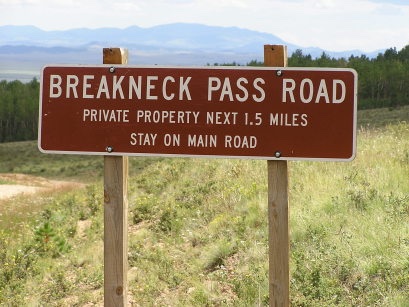This rectangular, landscape-oriented photograph captures a close-up view of a street sign. The sign, with a red background and white font, reads: "Breakneck Pass Road Private Property Next 1.5 Miles Stay on Main Road." It is mounted on two light brown wooden posts. The background features dry grass in shades of light brownish-green, dark green pine trees, and grayish-blue mountains in the distance. Overhead, a light gray cloud cover mostly obscures the skyline.